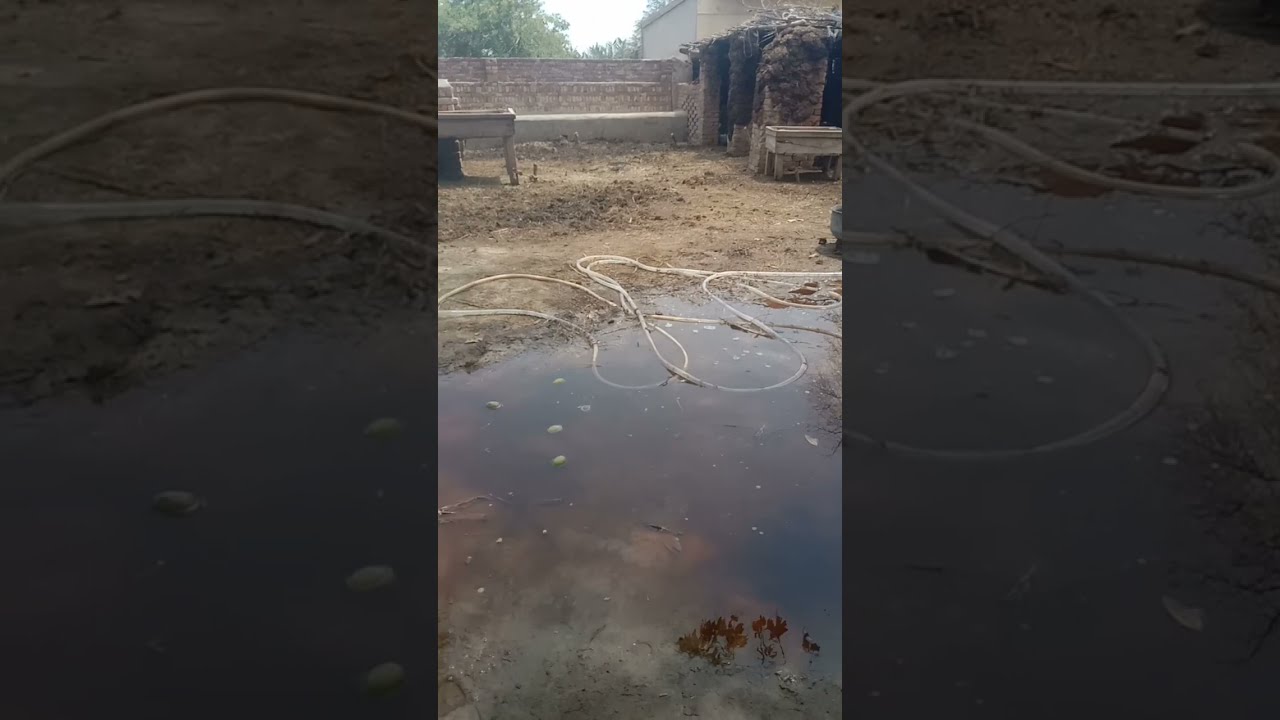The photograph, taken vertically with darkened, zoomed-in borders mirroring a portion of the image, depicts an untidy backyard or potentially a farm pen. The central focus is a dirty, brown puddle of water situated among a trampled, muddy dirt ground, surrounded by rubbish. A white rope, appearing to be part hose, lies partly on the dirt and partly in the murky water. In the upper right corner, there is a small structure, possibly a shed or boxed shelter area, topped with shrubs and leaves. Elements such as a table or large sink and the overall disorganized appearance suggest a lack of care for the area.